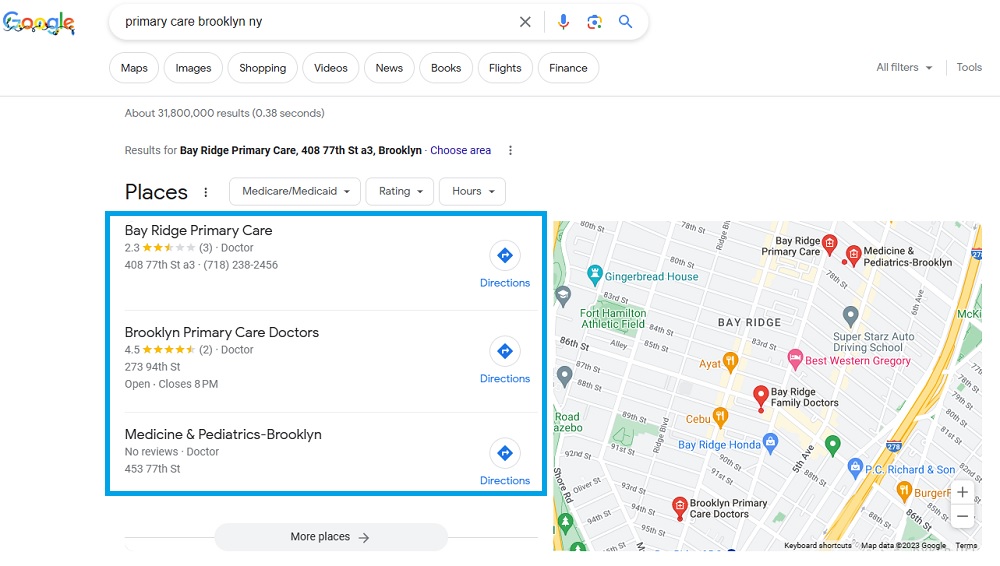This image is a screenshot of a Google search results page, displaying a themed Google Doodle in the upper left corner. The Doodle features the familiar Google logo embellished with whimsical, squiggly lines surrounding the letters, set against a white background. In the search bar at the top, the query "Primary Care Brooklyn, NY" is visible. Below the search bar, the navigation menu offers categories such as Maps, Images, Shopping, Videos, News, Books, Flights, and Finances, each framed by a subtle gray line.

The primary search results begin with a bold entry: "Results for Bay Ridge Primary Care, 40877 Street A3, Brooklyn." This is followed by a section titled "Places" encased in a blue-outlined, white rectangle. Three listings are provided: 

1. "Bay Ridge Primary Care" with a 2.3-star rating.
2. "Brooklyn Primary Care Doctors" boasting a 4.5-star rating, depicted with four full gold stars and a half-star.
3. "Medicine and Pediatrics Brooklyn," which has received no reviews.

On the right side of the page, a Google Maps snippet highlights the Brooklyn area, prominently marking the Bay Ridge neighborhood. Various location markers in blue, red, and orange are scattered across the map, pinpointing different notable places or services within the vicinity.